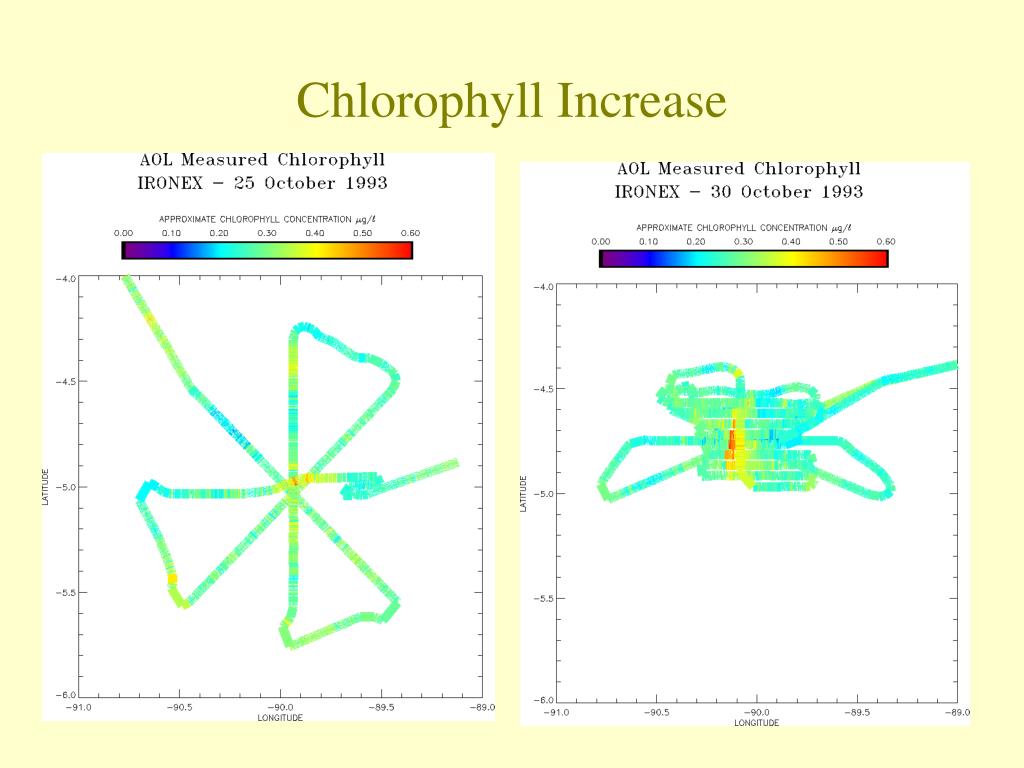The image depicts two detailed bar graphs or charts set against a light yellow background with white grounds for the graphs, focusing on the measurement of calligraphy increase, specifically regarding chlorophyll levels. At the top, labeled in green, are the titles “Chlorophyll Increase.” On the left chart, titled "AOL Measured Chlorophyll, Iron X-25, October 1993," a grid showcases a range of colors spanning from dark purple to bright red-orange, signifying chlorophyll concentrations from 0.00 to 0.60. This chart features a multicolored bar guide reminiscent of a rainbow, primarily displaying teals, greens, and yellows, and includes a shape formed by bluish and yellow lines within a table of latitude and longitude coordinates. The right chart, labeled "AOL Measured Chlorophyll II, Iron X-30, October 1993," mirrors the left but presents a more concentrated blue and yellow clump at the center, indicative of a different pattern in the chlorophyll levels.